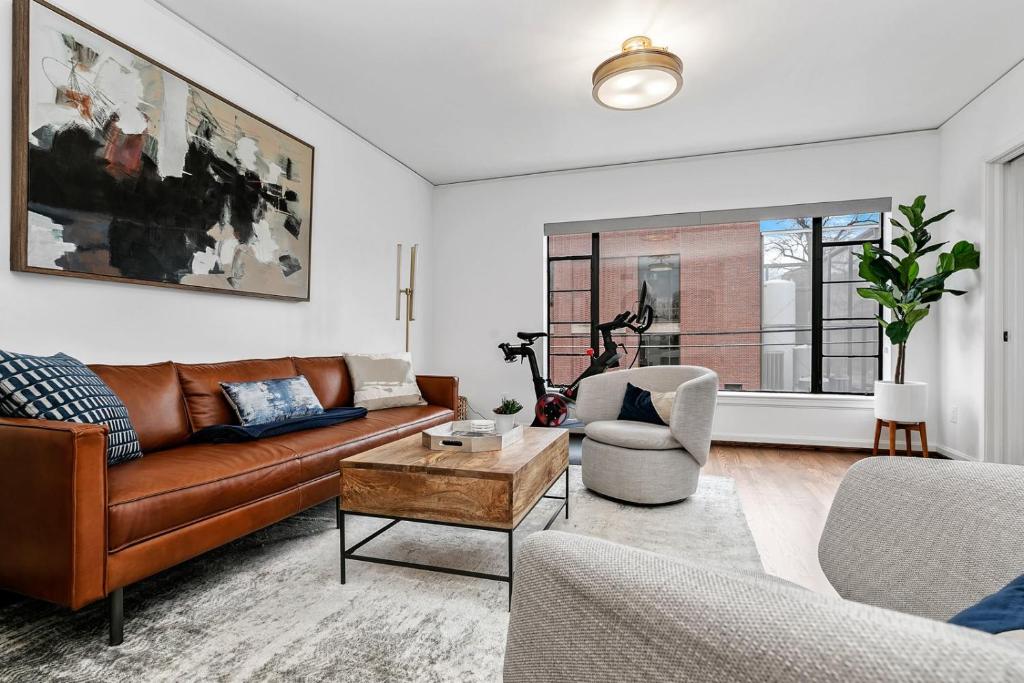A photograph depicts a modern living room with a white wall where a brown leather couch is set against it, displaying three distinct pillows: a black and white checker pattern on the left, a blue and white paint blotch pattern in the middle, and a light gray and white pillow on the far right. Above the couch hangs an abstract painting with black, white, and gray blotches. Directly in front of the couch is a coffee table featuring a black tabletop, wooden colored panels, and sturdy black metal legs. On the bottom right, part of a gray chair armrest is visible, adorned with a blue cloth. Central to the room, another gray chair with a circular backrest features a pillow split between white and black hues. Behind this chair sits a black exercise bike, oriented towards the right, next to a very large window with black frames. The window allows ample light, and balances the scene with the view of a neighboring brick building. In the upper right corner of the room, a vibrant green plant in a white pot rests on a wooden stool. The room’s decor is further illuminated by a ceiling light that casts a white and yellowish glow. The floor is wooden and beneath the central furniture, a white and gray rug enhances the cohesive aesthetic of the space.